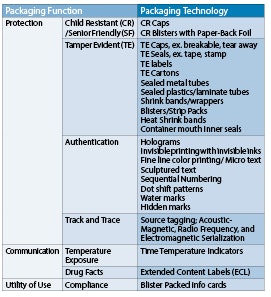The image is a detailed chart formatted like an Excel table, featuring various shades of blue, with lighter colors on the left and darker tones on the right. At the top left, the chart starts with a section labeled "Packaging Function," which is further divided into subsections. One subsection labeled "Protection" includes categories such as "Child-Resistant (CR)", "Sensor-Friendly (SF)", "Tamper-Evident (TE)", "Authentication," "Track and Trace," "Communication," "Temperature Exposure," "Drug Facts," "Compliance," and "Utility of Use." 

On the right side, the chart is divided under the heading "Packaging Technology" written in dark blue. This section lists different types of packaging such as "CR Caps," "CR Blisters with Paperback Foil," "TE Caps" (including examples like "Breakable" and "Tearaway"), "TE Seals" (with examples like "Tape," "Stamp," and "Labels"), "TE Cartons," and "Sealed Metal Tubes." Additional mentions include "Holograms," "Source Tagging," and "Time-Temperature Indicators."

Underneath the main sections, there are seven boxes, each in a different color. The boxes on the left side are lighter, transitioning to darker colors towards the right. The text in the chart is small, adding to the comprehensive yet compact presentation of the information. While the image quality is moderate, the chart effectively conveys detailed data about packaging functions and technologies.